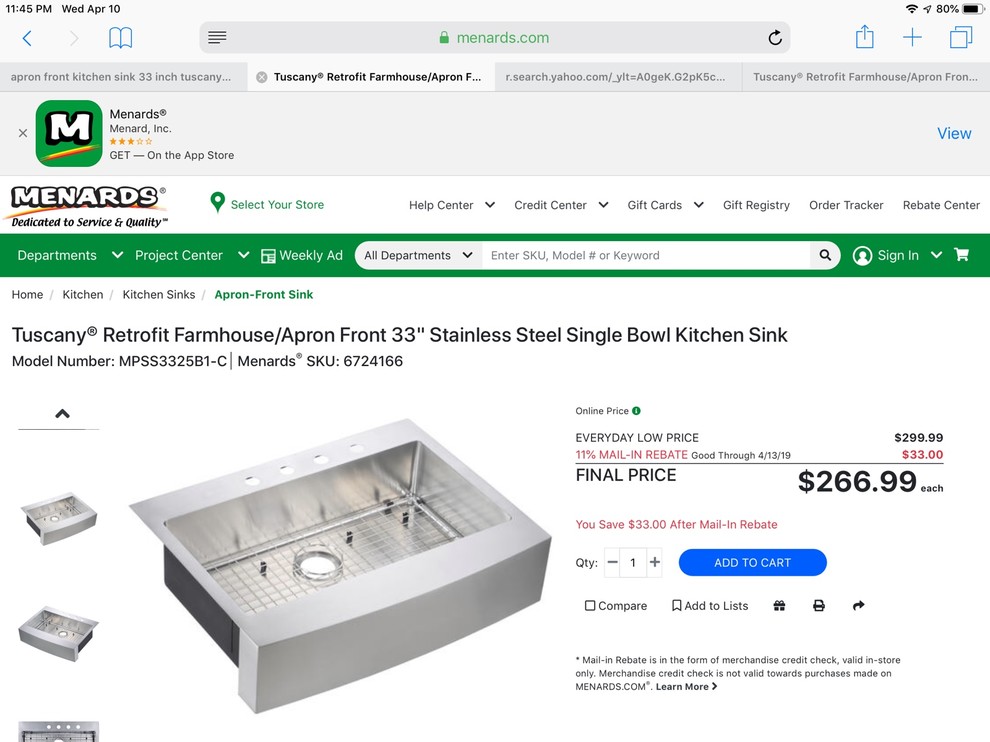**Caption:**

This image is a screenshot displaying a webpage from the retail website "maynards.com". The URL at the top is highlighted in green. The page features a product listing for a "Tuscany Retrofit Farmhouse/Apron Front 33-Inch Stainless Steel Single Bowl Kitchen Sink". The model number for this sink is listed as "MPSS3325B1-7" and the SKU number is "6724166". On the left side of the image, there is a clear photograph of the sink, showcasing its simple, sleek silver design. To the right of the photo, the listing indicates a final price of "$266.99 each".